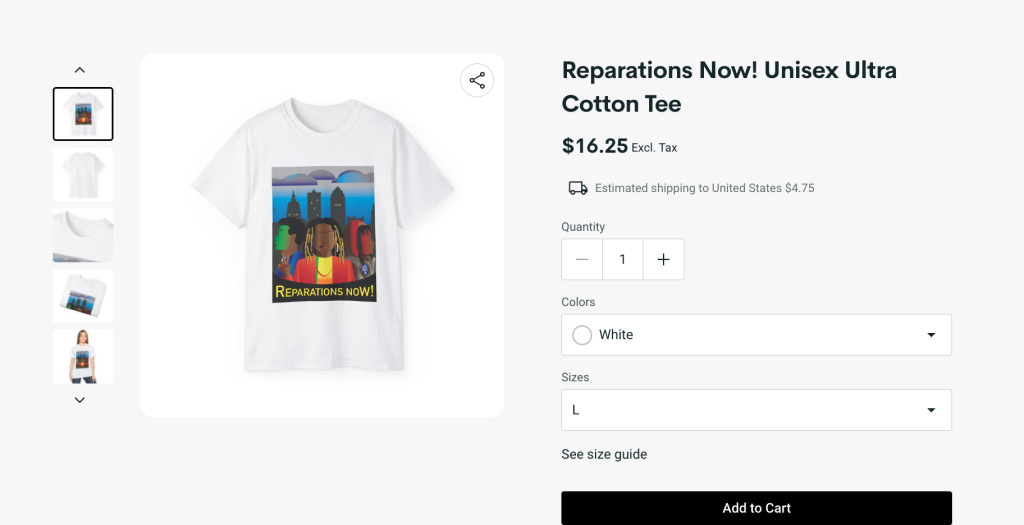White unisex ultra cotton t-shirt featuring a bold "Reparations Now" print. The shirt is available in size Large and the color white. On the back of the shirt, there's an intricate design set against a blue sky background, depicting the Twin Towers, the Grand Canyon with a sunrise, a large brown spaceship adorned with spaghetti, and a robot mask—the green one on the left and the red one on the right. Additional images include views of the shirt folded, the back design, and someone modeling it. Price estimate is $16.25 excluding tax, with shipping to the United States estimated at $4.75.